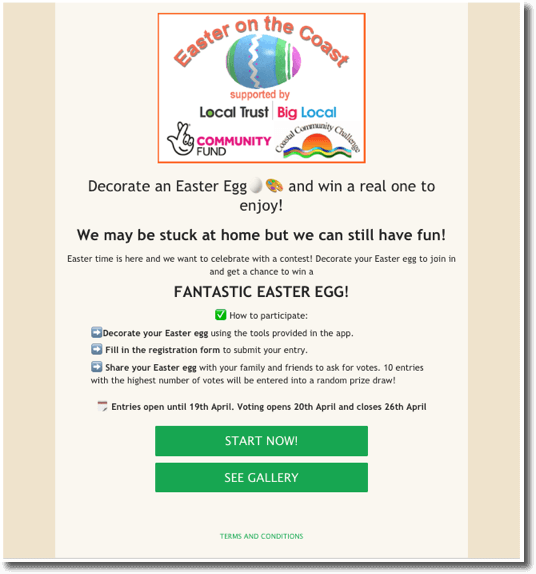**Descriptive Caption:**

The advertisement is a rectangular-shaped image primarily in shades of tan, with a lighter tan color in the center. At the top center, there is a small, intricately painted Easter egg in greens and blues with a white band in the middle, pink at the tip, and additional striping towards the top.

Above the egg, the event's name, "Easter on the Coast," is written in an orangish-red color. Below the event title, it states "Supported by," followed by "Local Trust" in black text. Adjacent to this, "Big" is displayed in pinkish-red writing, and "Local" in blue writing. Directly beneath these words, there is an outlined icon of a human hand with the index finger and middle finger crossed.

Next to this icon, the text reads "Community Fund," with "Community" in magenta and "Fund" in black. Nearby, an icon of an orange sunset is visible with the words "Coastal Community Challenge" written above it in black, slightly curved text.

The event description follows, explaining how participants can decorate an Easter egg to win a real one to enjoy. Below this description, two green rectangular buttons with white text are present. The top button says "Start Now," and the one below it reads "See Gallery." Further down, green text, which is a clickable link, reads "Terms and Conditions."